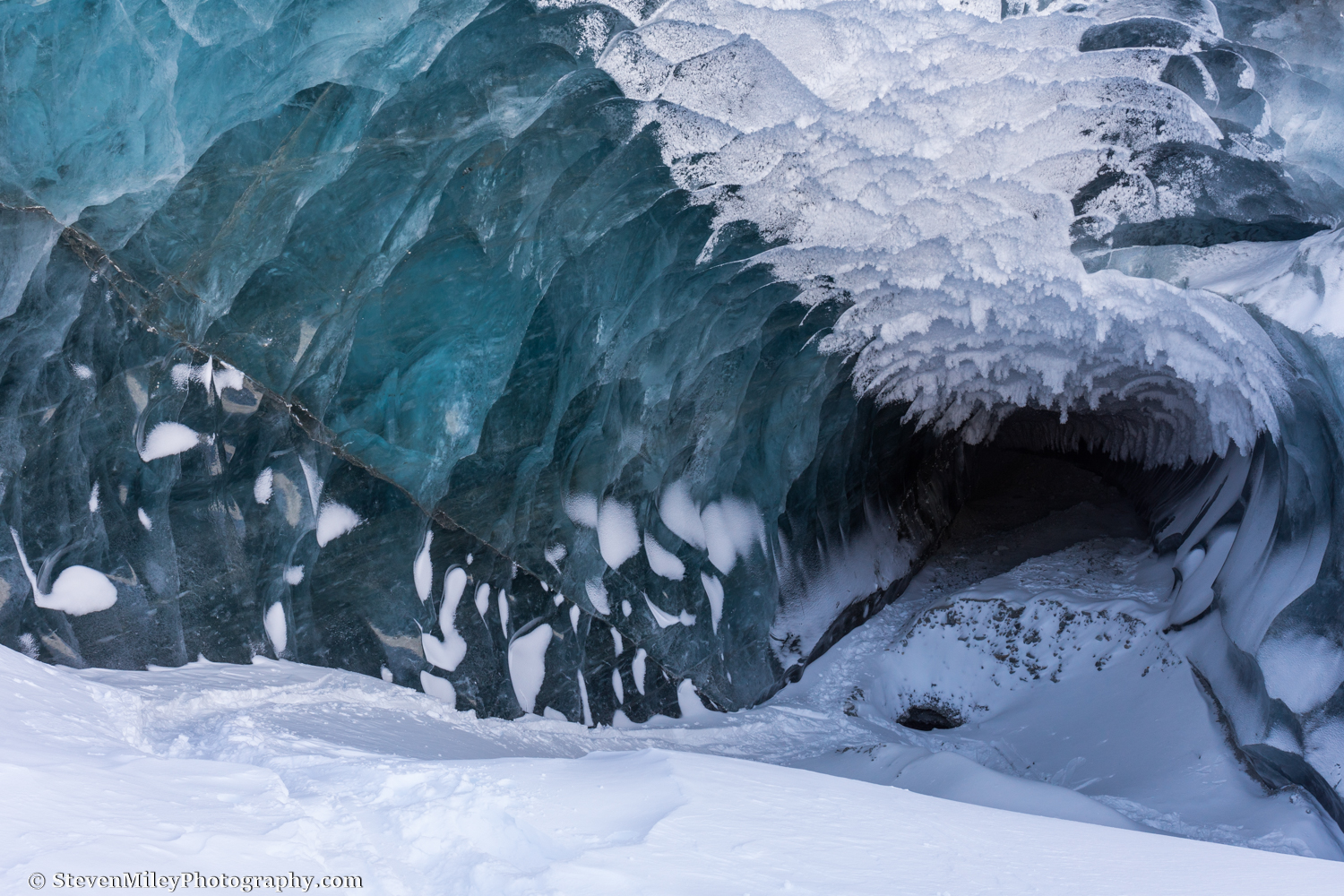This image captures a mesmerizing and potentially perilous cave entrance during winter. The entrance is carved into icy cliff walls, with snow partially covering the top. One side of the entrance showcases sheer, crystalline blue ice while the other is adorned with white ice crystals. Above the opening, there are overhanging snow formations that seem to be in a state of partial melt, yet frozen in a dripping shape. The ground is densely packed with snow, devoid of any footprints, suggesting the absence of animal activity. The icy entrance appears low and rounded, with a fissure originating from the upper left edge and cutting through the ice wall. The scene is both breathtaking and foreboding, with the cave interior shrouded in darkness, hinting at ancient and undisturbed depths. In the bottom left corner, the text "stevenmileyphotography.com" is visible.